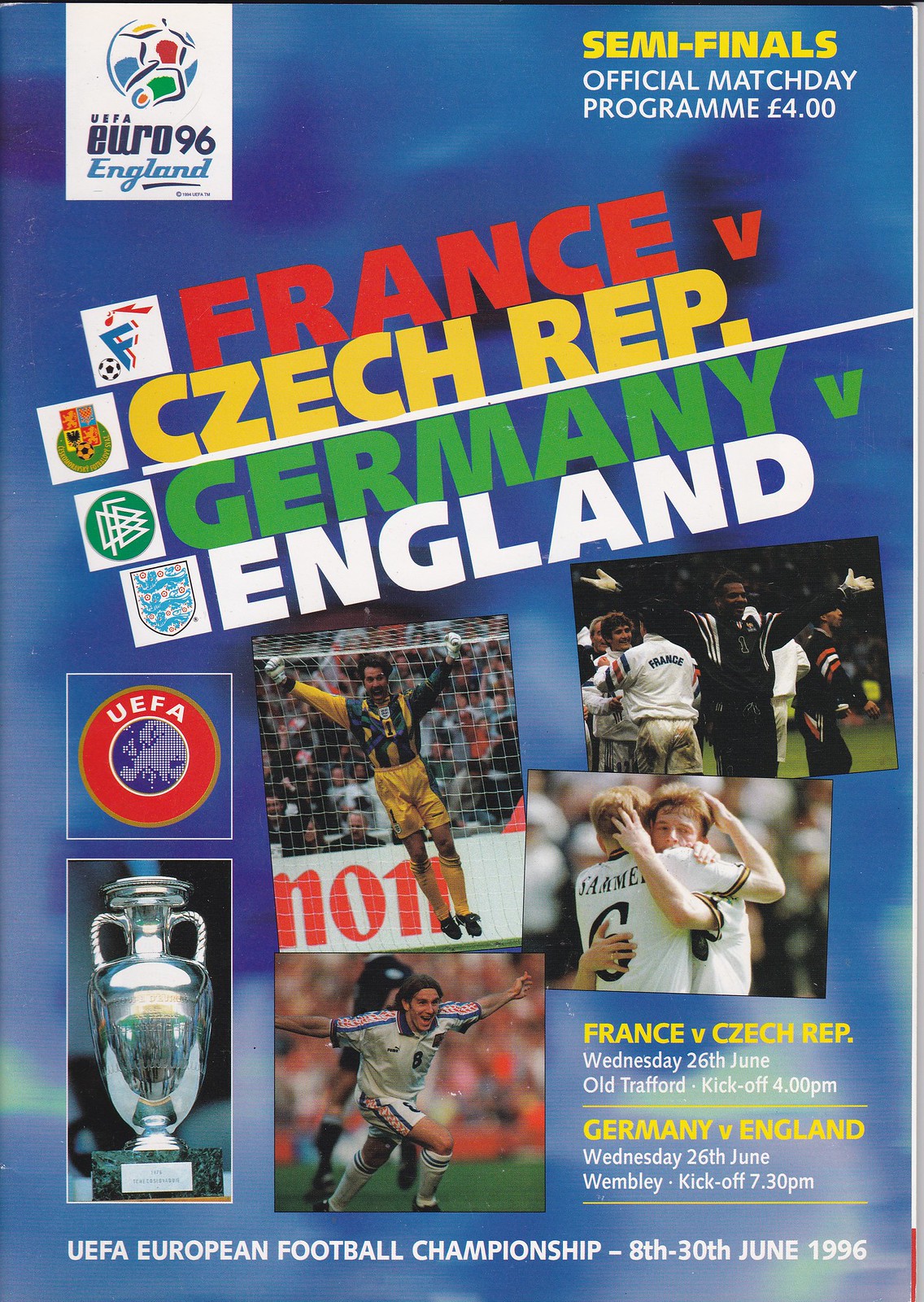This is a detailed program for the semifinal matches of the UEFA Euro 96 soccer tournament held in England. The background of the poster transitions from dark blue at the top to light blue at the bottom. In the upper left corner, there's a white square displaying a soccer ball adorned with blue, green, red, and yellow patches. Below the ball, it reads "WEFA Euro 96 England." In the upper right corner, "Official Match Day Program, Four Pounds" is written in white text. Positioned above this text, in yellow, it says "Semifinals."

Directly below in an angular style, the teams and match details are written: "France" in red followed by a "V," then "Czech REP." in yellow, followed by a period, separated by a white line from "Germany" in green followed by a "V," and "England" in white. 

In the central area, the images of key moments in the tournament are displayed. The central photo shows a goalie in mid-action, his hands aloft as he jumps off the ground, with the goal net visible behind him. This picture is overlaid with the orange letters "N O N" against a white background. Another image depicts a running soccer player with his hands outstretched. To the right of this sequence, the top image shows a black man in a black suit with his palms up in the air, soccer players visible behind him. Beneath this image, two players in white jerseys are captured in a celebratory hug.

Further text details the matches: "France vs. Czech Republic" in yellow, with the match date and venue, "Wednesday, 26 June. Old Trafford kickoff at 4 p.m." in white text. Below another yellow line: "Germany v. England" in yellow, with "Wednesday, 26 June. Wembley kickoff 7:30 p.m." in white.

The bottom of the program features the text: "UEFA European Football Championship - 8th - 30th June 1996." Situated in the bottom left corner is a picture of a silver trophy with two handles on a square base. Above this trophy, there's a red circle with "UEFA" written in white text, encircling a blue depiction of a pixelated Europe.